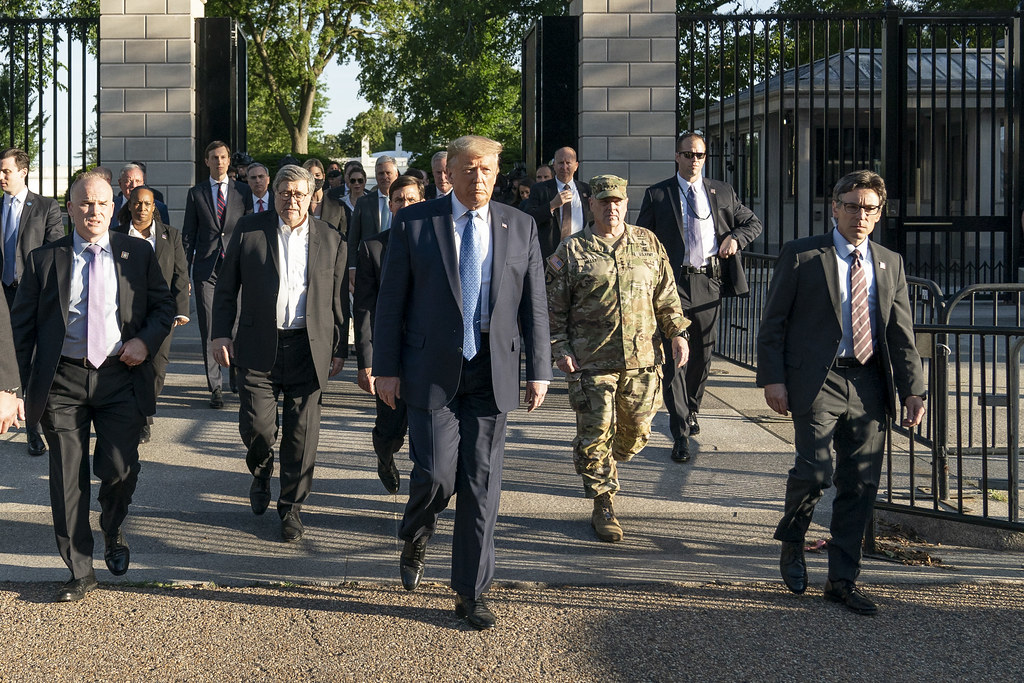In the photograph, President Donald Trump is prominently featured as he walks through a gated area, flanked by a group of men. Trump, wearing a blue suit, light blue shirt, and long blue tie, is at the center of the image. Directly to the right of him is a general in a brown army uniform, while to his left appears to be a heavyset man with curly hair, glasses, and a suit without a tie, who is likely his lawyer. Another man in a suit and tie is also close by. The background shows tan brick columns and a black wrought iron fence, suggesting they are exiting or entering a secure, institutional area. Surrounding Trump and the immediate entourage are several other men, some identifiable as security personnel by their attire and presence of flag pins on their lapels. The group is clearly in motion, walking with a sense of purpose, their destination or occasion unspecified.